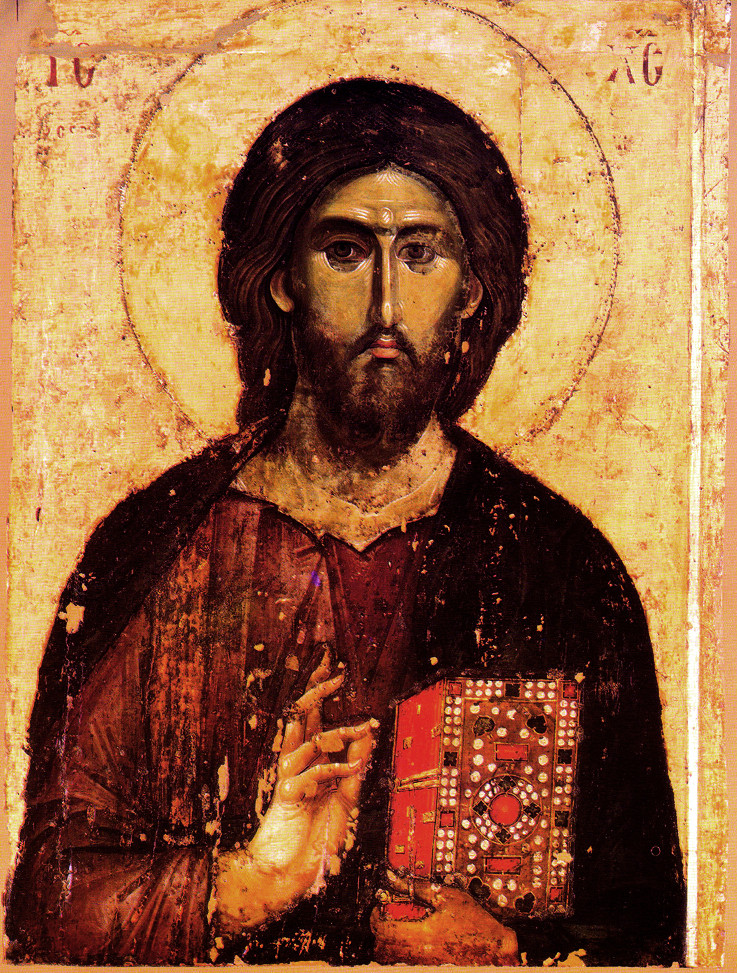This detailed painting vividly portrays Jesus as a religious figure, markedly identifiable by the halo encircling His head. He has long dark brown hair and a beard framing a contemplative face, with eyes slightly looking to the left. His expression is serious, with small, closed lips and a long, slim nose. His right hand is raised slightly above His chest, fingers open, possibly gesturing a blessing, while His left hand clutches a red book adorned with intricate black and white, or possibly golden, decorations. Jesus is dressed in dark robes with an additional garment draped over His right shoulder and covering the left side of His body. The background of the painting is a rich gold-yellow shade. Prominent in this backdrop are the initials "IC" and "XC" placed in the upper left and right corners respectively, suggesting a traditional iconographic portrayal. The letters in the upper left are partially obscured. Running through parts of the image is a subtle white line. This detailed composition indicates a profound religious significance, embodying a reverent and sacred representation of Jesus.